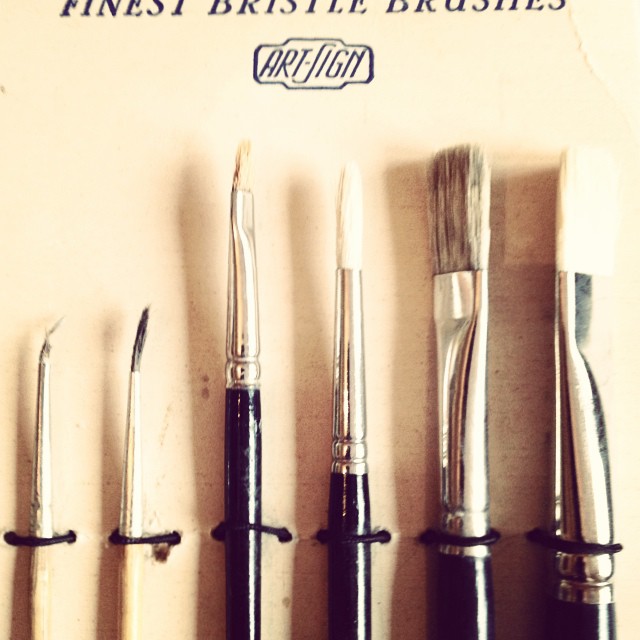The image depicts the packaging of artist paintbrushes against a light tan, cardboard-like background. The top of the packaging, partially cut off by the frame of the image, reads "Finest Bristle Brushes" in black text. Below this text is a rectangular logo that reads "Art Sign." The packaging showcases six paintbrushes, secured by a black string around their upper-middle sections. 

From left to right, the brushes transition from thin to thick. The first two brushes on the left have slender, cream-colored handles with silver ferrules; one has a white bristle tip and the other a black bristle tip. The middle two brushes have slightly thicker black handles; one has tan-brown bristles and the other has white bristles. The two brushes on the right are the thickest, also with black handles; one features light brown bristles and the other has white bristles. The photo captures the top and middle sections of the brushes, with the bottom portions cut off by the picture's frame.